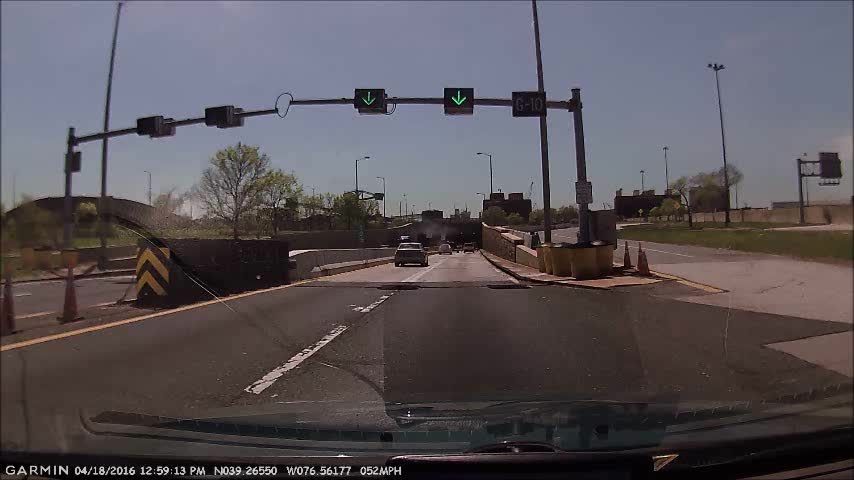This color photograph, captured from within a vehicle using a wide-angle lens, offers a slightly curved perspective from what appears to be a dashcam. At the bottom left corner, white text reads "Garmin" followed by coordinates and other details, indicating it's from April 18, 2016, at 12:59 p.m., with the vehicle traveling at 52 miles per hour. The image shows a grey road with a white line running down the center, which lightens as it extends into the distance.

In the foreground of the road, several vehicles are visible, including a silver sedan. The road appears to be part of a one-way highway, under an overpass, with a blue but muted sky overhead. On the left, an unbroken grey barrier features a yellow and black diagonal warning sign at its end. On the right, a lighter-colored wall runs parallel to the highway, leading to an exit lined with grass, small trees, larger street signs, and electricity poles. 

Two poles on either side of the road support traffic signs that intersect in the middle, displaying green downward-facing arrows and a rectangular “G10” sign. In the far distance and center of the photograph are additional lighting poles, reinforcing the structured and utility-driven environment of this stretch of roadway. To the left background, there is a building and some trees, whereas to the right, utility poles and another type of sign are present.